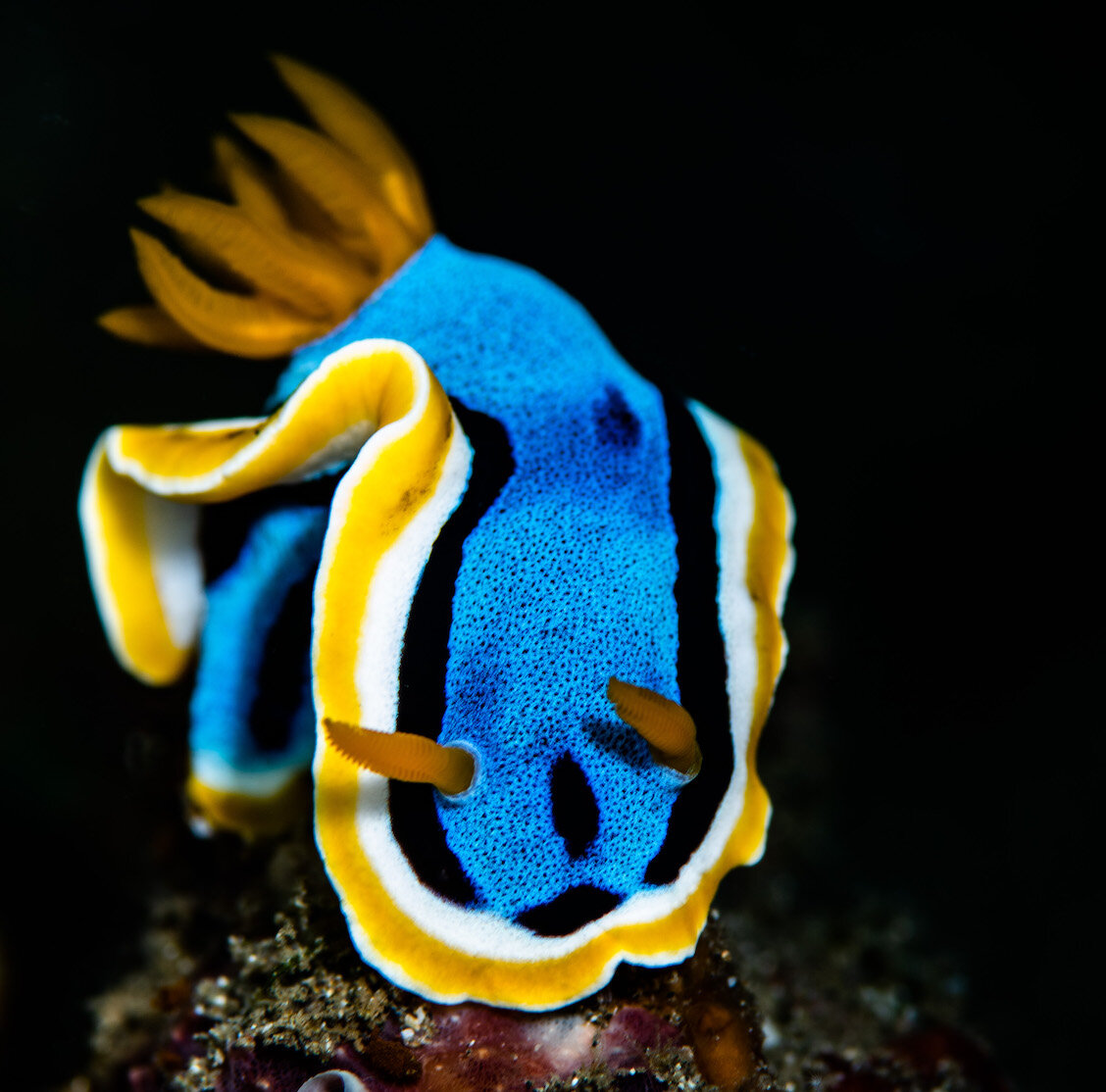The photograph depicts a vividly colorful sea slug, potentially a type of nudibranch, situated in its natural underwater habitat. The slug’s elongated, wavy body showcases a striking array of stripes: a light blue central stripe adorned with tiny black spots, bordered by sequential bands of black, white, and yellow. Adorning the edges of its ruffled body are vibrant yellow accents. The face of the slug is directed towards the camera, revealing two distinctive dark yellow, brush-like antennae curving slightly to the left. At the rear of the creature, several thin, dark yellow projections resembling small, delicate tentacles or peach wedges emerge. The surface on which the sea slug rests appears textured and varied in color, with splotches of white, orange, and purple, resembling barnacles or coral fragments. The backdrop of the image is entirely black, emphasizing the intricate details and vivid colors of the sea slug and its immediate surroundings.